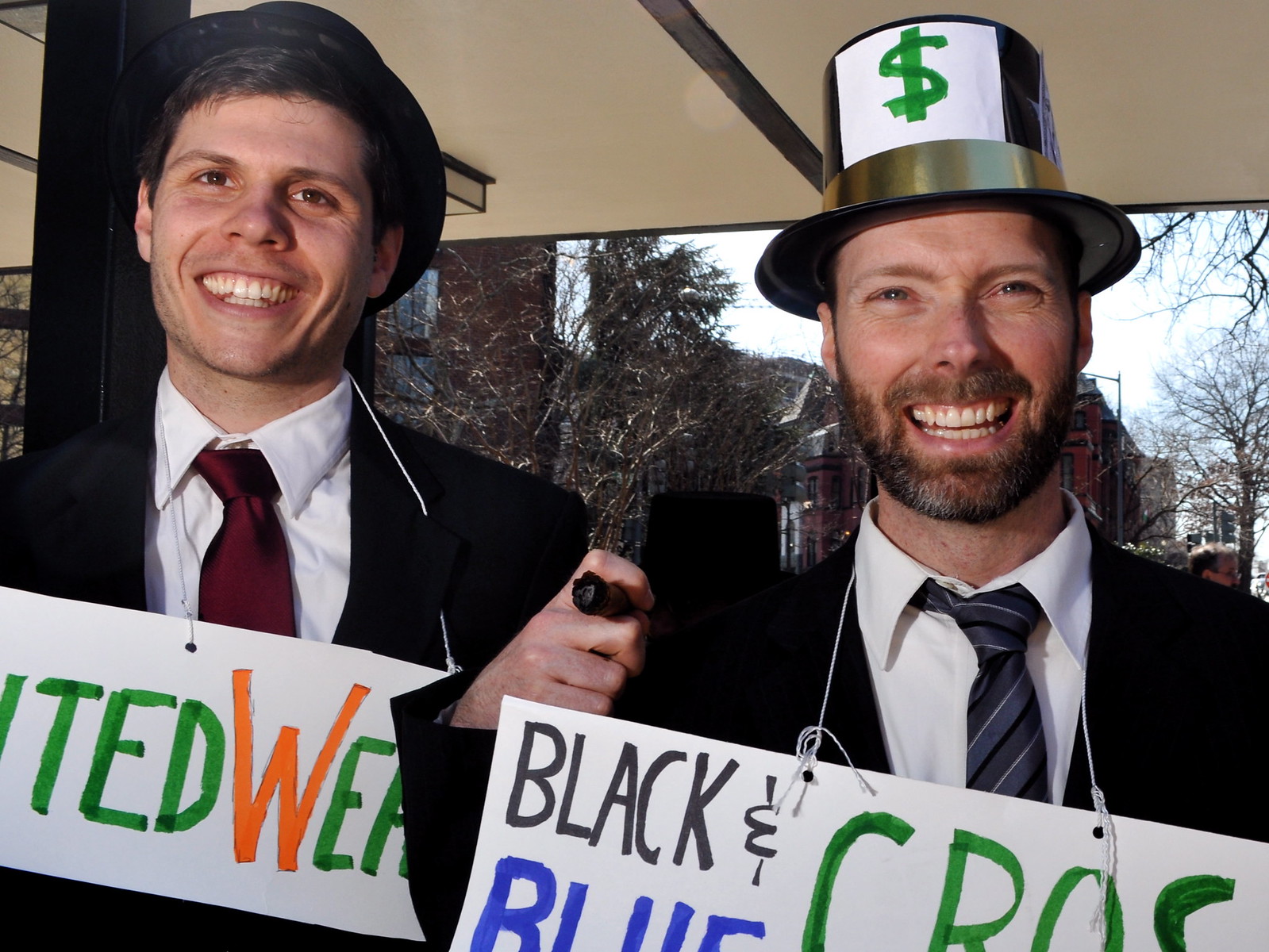In this close-up photograph, two smiling men, both wearing black suits and white dress shirts, pose for the camera. Each has a sign hanging from their necks. The man on the right, who has a beard, sports a black plastic top hat adorned with a piece of paper displaying a green dollar sign. He wears a light gray and black striped necktie and his sign, secured by a string around his neck, reads "black" in black text, "blue" in blue text, and though partially obscured, likely continues with "Crocs" in green text. The man on the left, clean-shaven, wears a short black top hat and a red necktie. His sign, also on a string, prominently shows "Ted" in green text, "W" in orange text, and partially visible letters "EA". Both men are framed against what appears to be an outdoor setting, possibly under a tent or awning. The right man also holds a cigar, adding a casual touch to their formal attire.